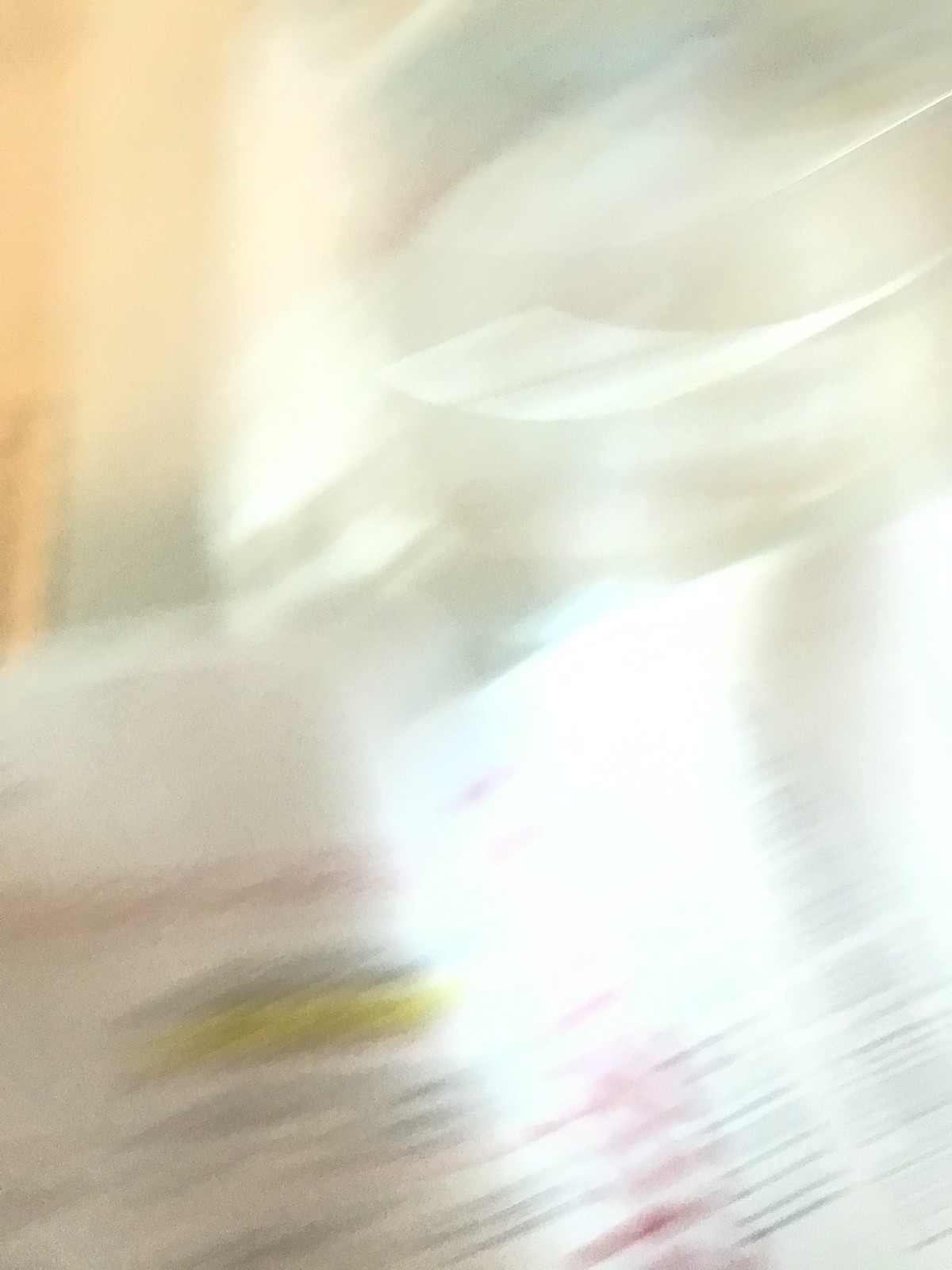This extremely blurry photograph captures a chaotic and unintentionally taken image, possibly a pocket shot. Dominated by a hot white center, the picture shows no decipherable subject due to the rapid movement of the camera, which creates a diagonal, horizontal stream of light. Hints of red, yellow, and various shades of gray blend into the chaotic scene, with streaks and darker lines integrated within these colors. The upper left-hand corner features a tan or peach-colored surface that might resemble a wall with the edge of a doorway. This organic, white shape of light in the top part of the image suggests a flash might have gone off, adding to the overall flat and dimensionless appearance. Amidst the blur, there's a perception of white printed material, such as a menu or newspaper, and possible outlines of a person's head in the upper right, all contributing to the image's unplanned and frenetic composition.